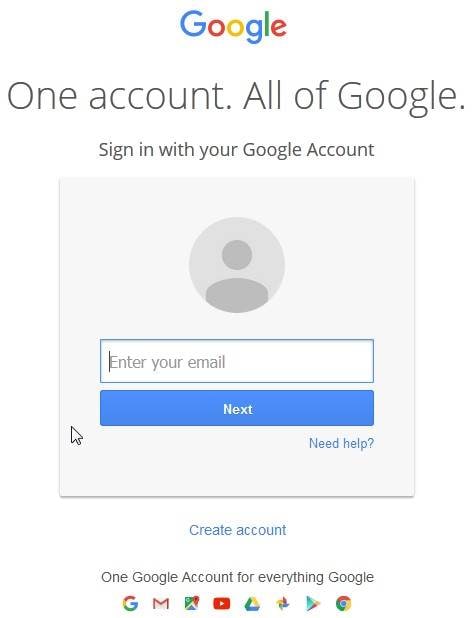The image showcases a Google sign-in page with the heading "One account. All of Google." prominently displayed at the top. Below the heading, there is a prompt that reads, "Sign in with your Google Account.”

At the center of the page, there is an empty text field labeled "Enter your email,” inviting users to input their email addresses. Directly beneath this field is a blue button that spans the same width as the text field, designed for users to proceed after entering their email.

To the bottom right of the text field, the phrase "Need help?" appears in blue, accompanied by a question mark. Just below this, there is a small square icon containing a circle with a stylized person icon in dark gray against a lighter gray background.

Underneath this icon, the "Create account" option is highlighted in blue. The phrase "One Google Account for everything" follows, alongside several recognizable Google icons, including those for Google, Gmail, Maps, YouTube, Google Drive, Photos, Play Store, and Google Search.

The entire layout is set against a clean, white background with color elements in red, yellow, green, blue, black, and gray. The primary interactive element, the text field for email entry, features a subtle drop shadow on its bottom and left sides, giving it a slight three-dimensional effect.